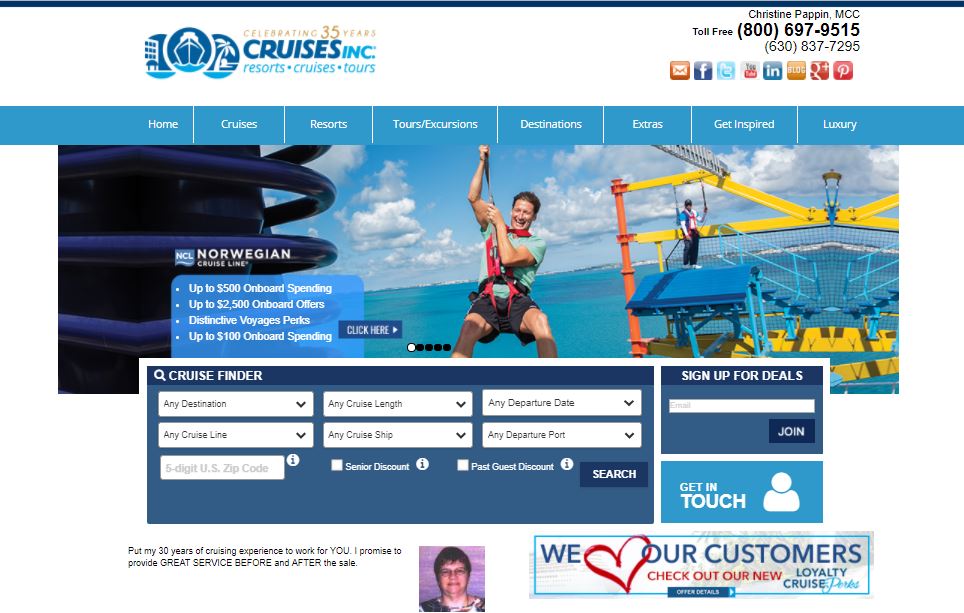**Caption:** 

The image depicts a detailed webpage celebrating the 35th anniversary of Cruises Inc. At the top, the headline reads "Celebrating 35 Years," adorned with icons representing a resort, a blue cruise ship, and a beach scene with a white palm tree. The webpage is hosted by Christine Pappin, MMC, with contact numbers toll-free at 800-697-9515 and 630-837-7295 listed prominently. Social media icons for Facebook, Twitter, and YouTube, among others, are displayed below her contact information.

Navigation tabs span the page, offering links to Home, Cruises, Resorts, Tours and Excursions, Destinations, Extras, Get Inspired, and Luxury. Below the tabs, a promotional section highlights offers from Norwegian Cruise Line, including up to $500 in onboard spending and up to $2,500 in onboard offers, with "Distinctive Voyage Perks" providing an additional $100 onboard spending. A vibrant "Click Here" button is seen next to an image of an exhilarated man zip-lining against a lively yellow and orange backdrop, where another person prepares for an adventurous activity.

The page features a Cruise Finder search function where users can enter preferences such as Destination, Cruise Length, Date, Cruise Line, Cruise Ship, Departure Port, and Zip Code. There are options to tick boxes for a Senior Discount or a Past Guest Discount, followed by a blue search button.

Additionally, a "Get In Touch" section is present, emphasizing Christine Pappin's 30 years of cruising experience with a promise to deliver excellent service before and after the trip. Her image is displayed, and the bottom corner of the page features a message encouraging customers to check out the new Loyalty Cruise Perks, highlighting the company's commitment to customer satisfaction.